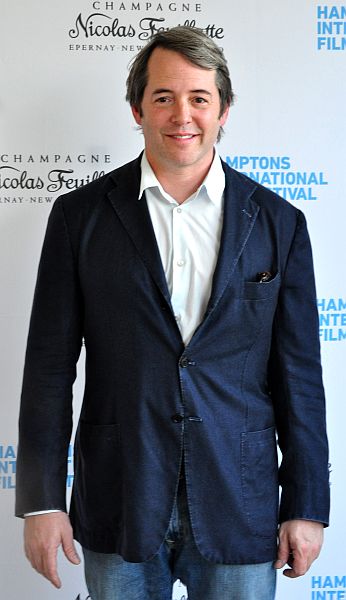The image showcases actor Matthew Broderick standing in front of a light blue backdrop adorned with multiple repeating logos. Broderick, who appears to have a mix of brown and silver hair slicked to the side, and a receding hairline, is smiling directly at the camera. He is wearing a white button-down collared shirt, layered under a blue blazer, with blue jeans. A black item is visible in his breast pocket. The backdrop text includes partially obscured names and phrases such as "Champagne Nicolas Feuillatte," "Epernay New York," and "Hampton's International Film Festival," though some letters are cut off. Broderick's attire and pose convey a neat and happy appearance.